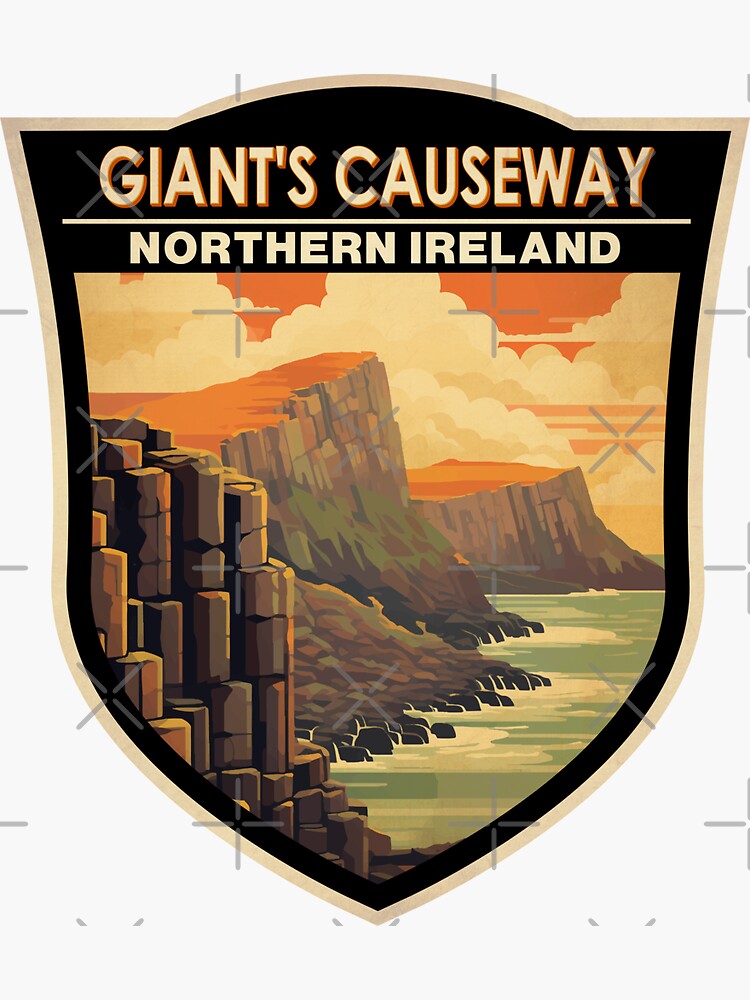The image is a detailed, digitally-created badge depicting the Giant's Causeway in Northern Ireland. Shaped like a badge, it is outlined in tan with an inner black border. At the top, the words "Giant's Causeway" are prominently displayed in cream and outlined in orange, set against the black background. Below the text, the words "Northern Ireland" are written in all capital letters, also in cream. Underneath this, a horizontal cream line separates the text from the central graphic. The main image is a stylized illustration of the Giant's Causeway, featuring a landscape of jagged, brown cliffs with patches of green moss and burnt orange tops, evoking the iconic basalt columns. The background sky is a striking burnt orange with puffy cream clouds. Black rocks are scattered around the coastline where the cliffs meet the sea, adding to the rugged appearance of the scene. The badge's design suggests an advertisement for the scenic Northern Irish landmark.